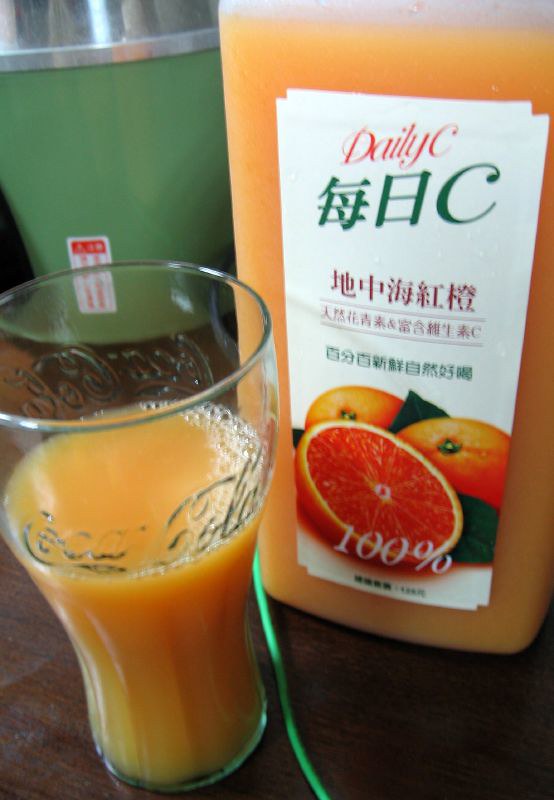In this indoor image, the scene is quite compact and features a brown wooden table or countertop. In the background, a green bowl with a silver interior is positioned, adding a subtle splash of color. Dominating the foreground is a distinctly recognizable Coca-Cola glass, with the iconic Coca-Cola logo etched into it. This glass exhibits the classic design, being narrow at the bottom and gradually widening towards the top. Adjacent to the Coca-Cola glass lies a green cord, likely a charger of some sort. Positioned beside the Coca-Cola glass is a bottle of juice labeled "Daily C," displaying this text in three different languages. The bottle proudly declares "100%" and showcases images of oranges, complementing the orange juice that fills the glass.